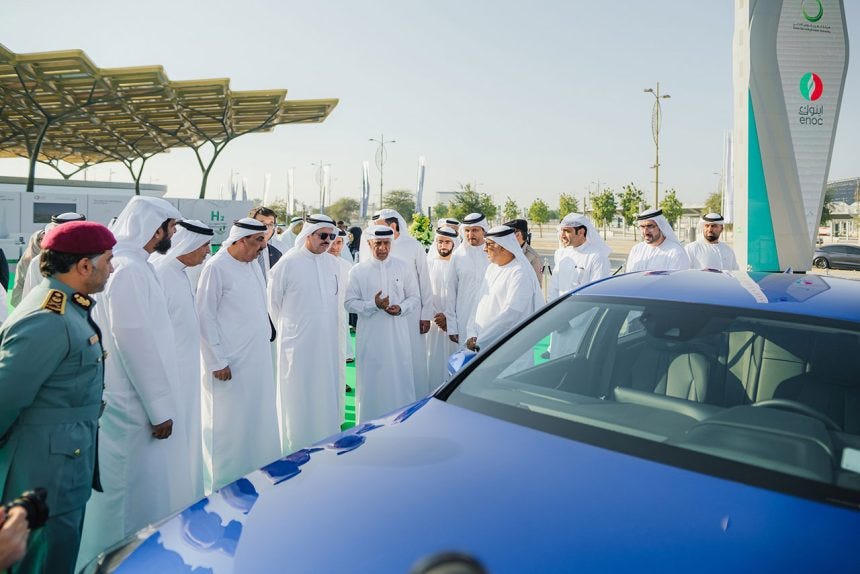The image shows a group of Middle Eastern men, predominantly dressed in traditional white robes and white headscarves secured with black bands, commonly associated with Saudi Arabia and Dubai. The focus is on a blue sedan car in the foreground, which they appear to be examining and discussing with great interest. Among the group, there is a notable exception – one man in a military uniform with a red beret. The men are gathered under a shade structure supported by stylized, tree-like metal pillars. The backdrop features a clear bluish-white sky and text displaying "H2," suggesting that the car might be a hydrogen-powered vehicle. The scene hints at a significant unveiling or demonstration of this new automotive technology.